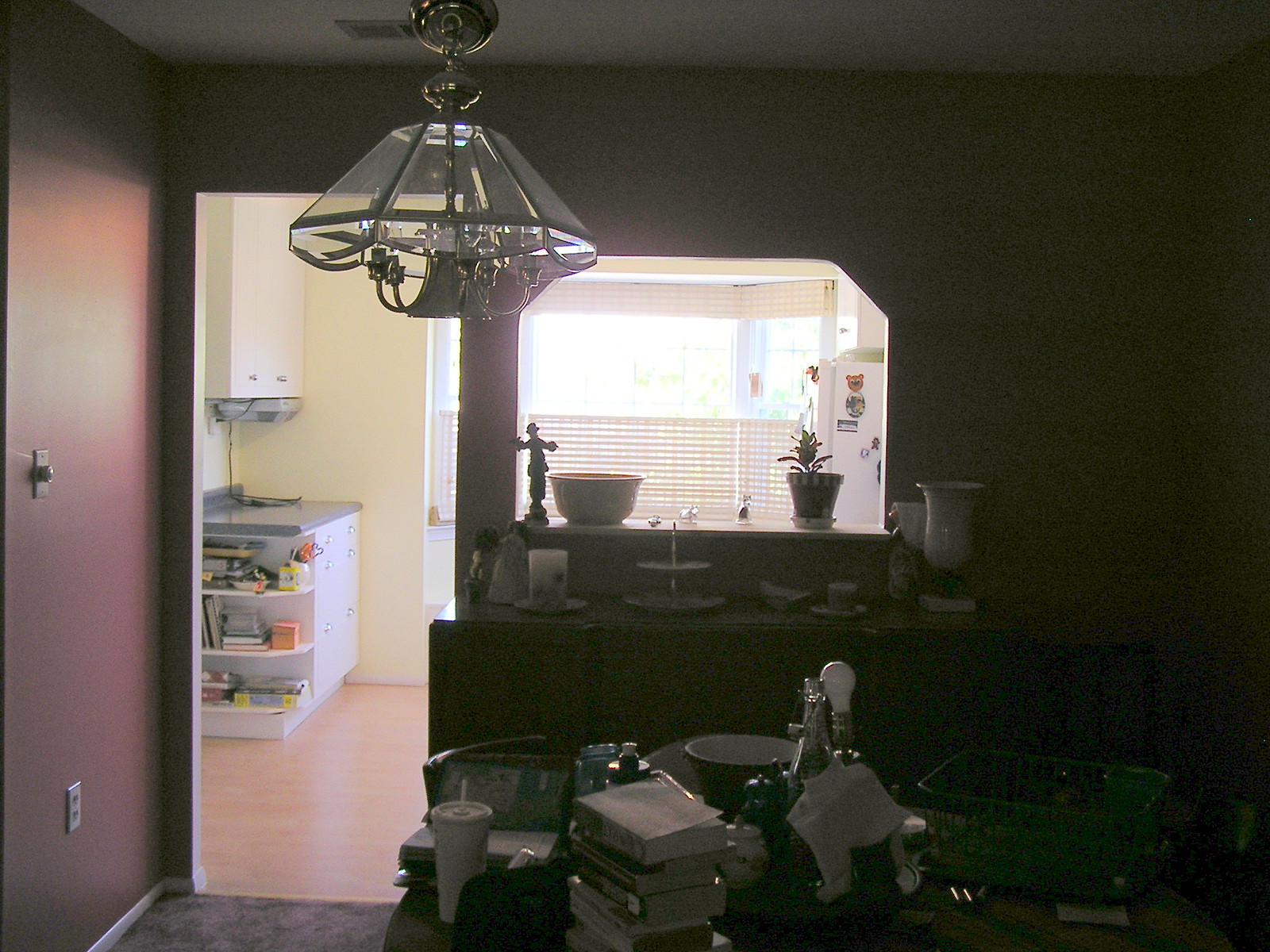The dimly lit dining room features red walls and gray carpet. Dominating the center is a cluttered dining table, laden with various items: tall stacks of paperback books, a green dish basket, a lamp without a shade exposing a white light bulb, a foil-wrapped bottle, a green bowl, and a large white cup alongside an open book. To one side stands a brown hutch displaying large vases and a tiered stand for cakes and candies. A broad pass-through window showcases a plant, a large white bowl, and a small statue. Beyond, the kitchen reveals a large open window with shades drawn halfway, the top of a white refrigerator visible. Adjacent to it is a small cabinet, a long white cabinet on the wall, a bottom cabinet, and an end shelf filled with books and papers.